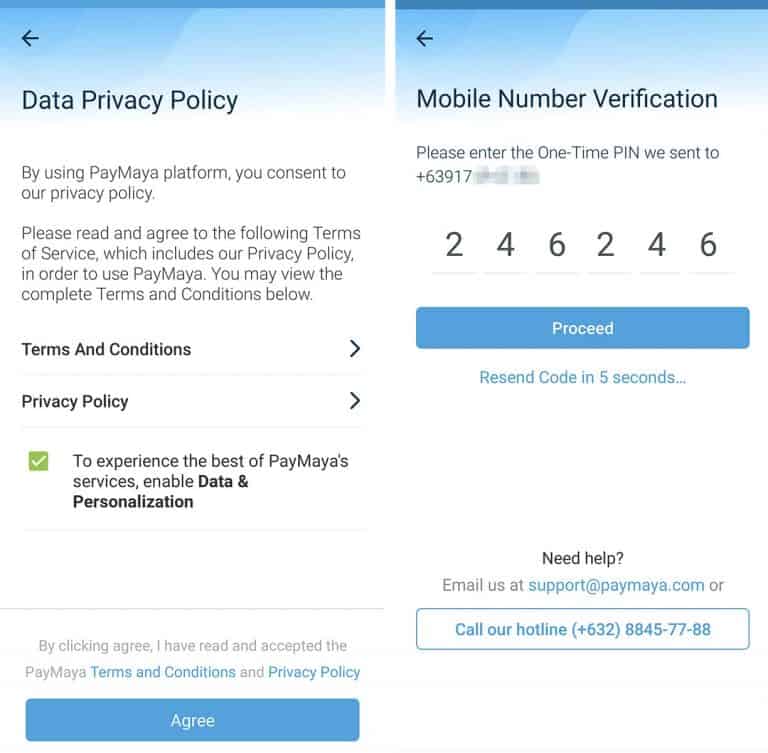The image consists of two mobile phone screenshots positioned side by side. 

On the left screenshot, the top section displays a blue cloudy sky graphic. Below this graphic, in black font, the heading reads "Data Privacy Policy." The rest of the page is white, featuring black text that states: "By using PayMaya platform you consent to our privacy policy. Please read and agree to the following terms of service, which includes our privacy policy. In order to use PayMaya, you may review the complete terms and conditions below." Two dropdown menus are provided: one labeled "Terms and Conditions" and the other "Privacy Policy." Further down, it advises users to "Enable Data and Personalization for the best PayMaya experience," which has been selected. In gray font, there's a declaration: "By clicking 'Agree,' I have read and accepted the PayMaya terms and conditions and privacy policy." Below this text is a button labeled "Agree."

The right screenshot mirrors the same blue cloudy sky graphic at the top. Underneath, the title reads "Mobile Number Verification" in black font. The instructions below, also in black, ask the user to "Please enter the one-time PIN we sent to +63917," with the rest of the number blurred out for privacy.